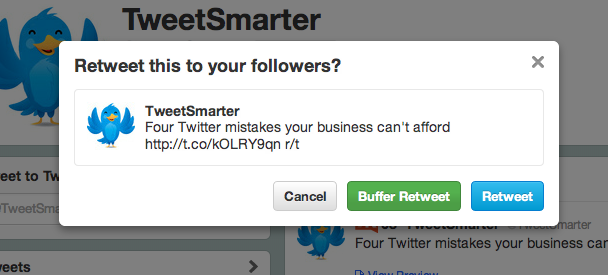This is a screenshot of a website called "Tweet Smarter". The focal point of the image is a cheerful illustration of a small, happy bird raising its wings. Accompanying the bird is a pop-up box with the text: "Retweet this to your followers? Tweet Smarter for Twitter mistakes your business can't afford." The pop-up box presents three clickable options labeled "Cancel," "Buffer Retweet," and "Retweet." 

The "Cancel" option allows users to dismiss the action. "Buffer Retweet" seems to refer to scheduling the retweet for a later time or date through a service like Buffer. The "Retweet" option enables immediate sharing of the tweet with the user's followers.

The image appears to be promoting "Tweet Smarter," an app designed to help businesses optimize their Twitter activity. This includes making strategic retweets and scheduling posts to maximize engagement. Due to the outdated Twitter interface in the background, it is unclear whether "Tweet Smarter" is an older platform or if the screenshot is from a previous version of the website. Nonetheless, it implies that "Tweet Smarter" assists businesses by advising on Twitter best practices and timing for posts.